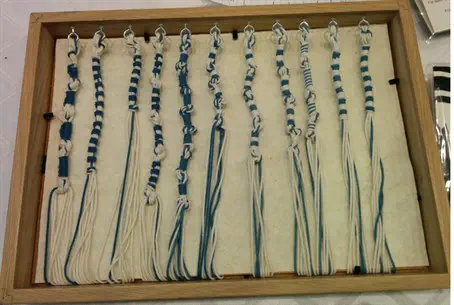The image depicts an open wooden box with visible wood grain on its sides, creating a natural brown frame. Inside the box, there is a cloth lining, possibly white or cream in color, serving as a background. Arranged neatly on the cloth are several handmade friendship bracelets. The bracelets, crafted from yarn in blue and whitish-gray hues, feature intricate details such as braids, beads, and silver clasps. Some of the bracelets have tassels hanging down, and the yarn appears to have been expertly woven into various stripy patterns. The overall composition highlights the craftsmanship of the bracelets against the simple, rustic backdrop of the wooden box.